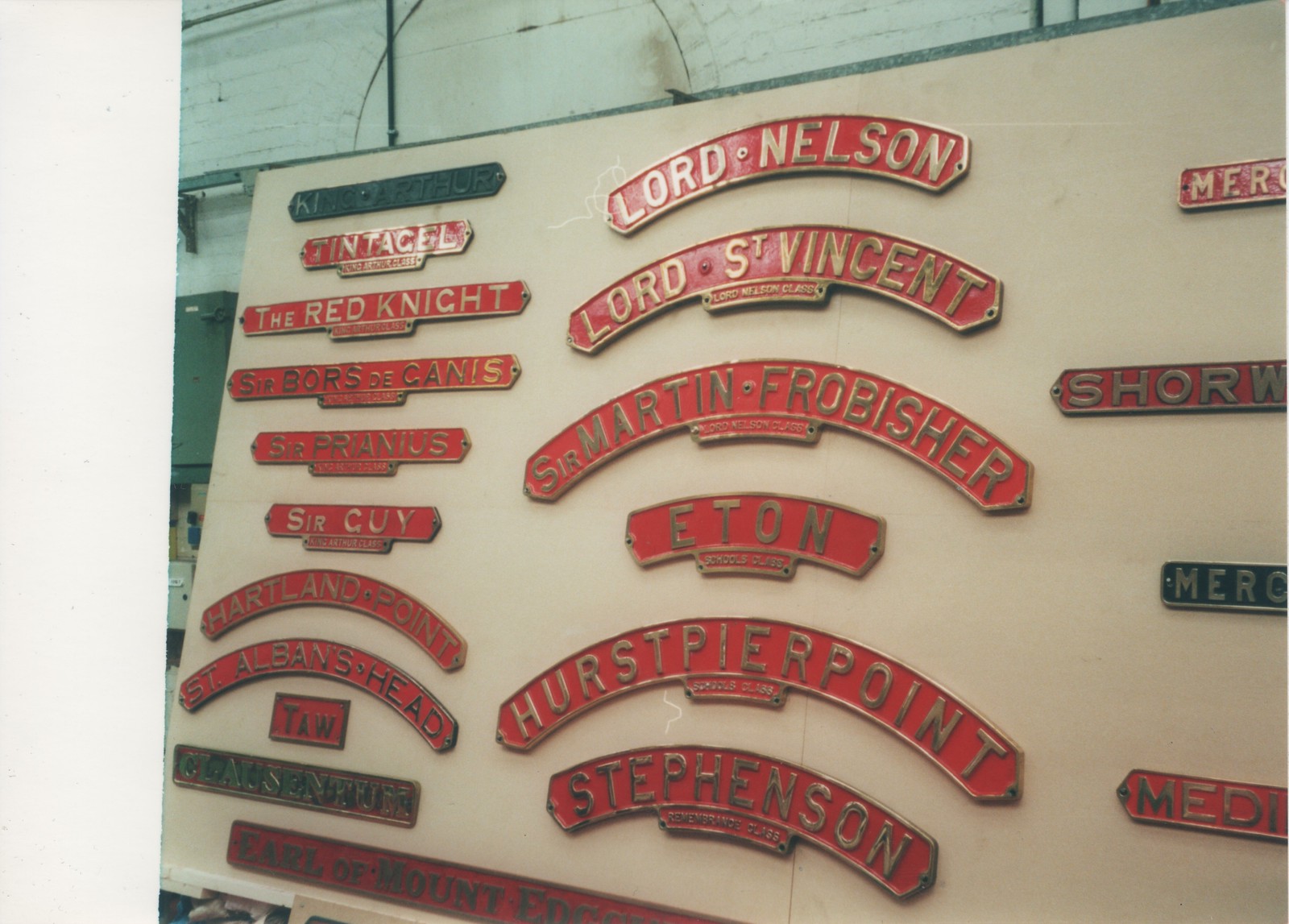The image depicts a large signboard set against a white building with dark gray trim, featuring numerous nameplates affixed to a light brown wooden board. The background is characterized by a large metal wall, with a green lower half and a lighter green upper half. The nameplates are predominantly red with gold lettering, though there are a few green ones as well. In the very upper left corner, a faded green nameplate appears to possibly read "King Arthur." Another notable green nameplate, located second from the bottom on the left, has partially gold ends and seemingly reads "Glaucentum," while a similarly green and silver nameplate lower on the left reads "M-E-R-O" though the rest is cut off. In the middle of the board, a red semicircular nameplate with gold letters says "Lord Nelson," followed by another red nameplate with gold text reading "Lord St. Vincent." Additional names like "Sir Martin Frobisher" and multiple others such as "Eaton" and "Hearst Pier Point" and "Stevenson" are also visible in the red and gold format. The nameplates are a mix of new and weathered, with some being curved and others straight. The composition includes a few blue nameplates with white or gold text and an overarching red banner with gold lettering partially cut off at the bottom of the photo.